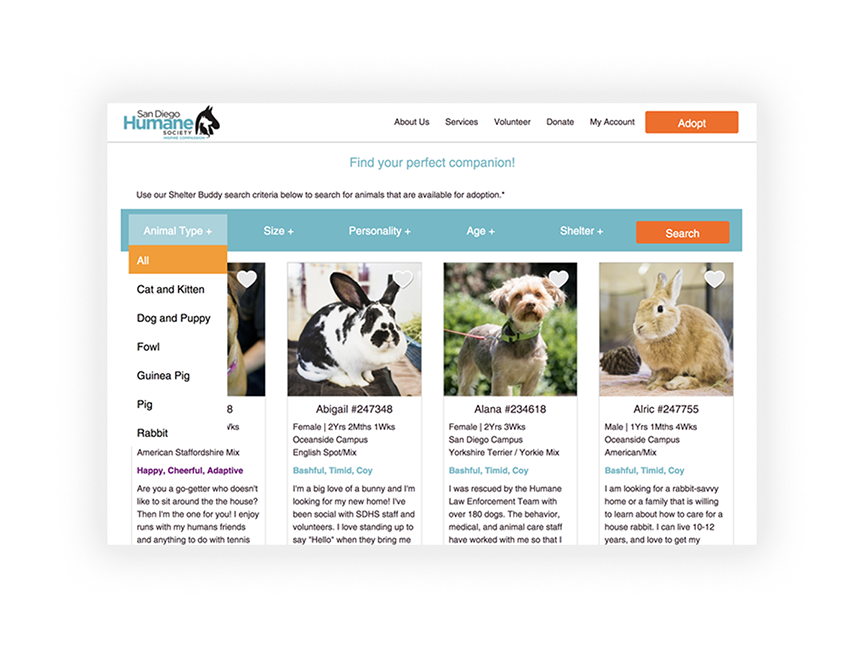This image is a detailed screenshot from the San Diego Humane Society's website. The organization’s logo, featuring interposed animal silhouettes in black and blue, is prominently displayed in the top left corner against a white horizontal bar. Adjacent to the logo on the right are navigation links labeled About Us, Services, Volunteer, Donate, and My Account, along with an orange rectangular box containing a hyperlink for Adopt.

Centered below this navigation bar, the heading in blue text invites users to "Find Your Perfect Companion." It is followed by a subheading that encourages users to utilize the "shelter buddy search criteria below to search for animals that are available for adoption." A light blue horizontal bar beneath this offers filtering options for different categories of animals. The currently hovered category, "Animal Type +," expands to reveal filter options such as All, Cat and Kitten, Dog and Puppy, Fowl, Guinea Pig, and Rabbit. Other filtration categories include Size, Personality, Age, and Shelter, along with another orange rectangular box for the Search hyperlink.

Further down, the user can see various animal profiles displayed with corresponding pictures: the first with a partially visible dog, the second and fourth showcasing rabbits, and the third featuring another dog. The layout is designed to help users efficiently navigate through available animals for adoption.